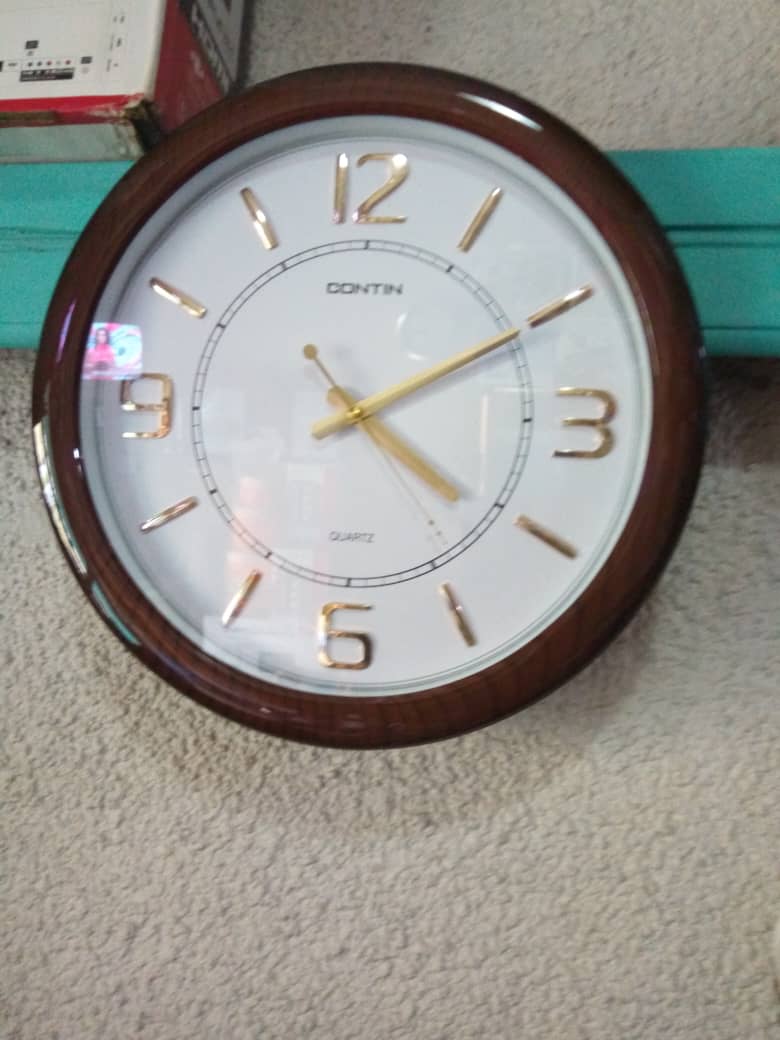The image depicts a round, basic clock placed on a carpeted floor, not mounted on a wall. The clock face is dark brown with a glass cover that shows a glare from the side. Gold-colored hands and numbers—specifically, the 12, 3, 6, and 9 hours—are clearly visible, while lines replace the other hours. The time displayed on the clock is 4:10, with the second hand around 19 seconds. The clock's hour, minute, and second hands are also gold. The strap of the watch is turquoise. Surrounding the clock, the background appears white and bumpy, and a box can be seen in the top left corner. The box features a white front and red and black sides with white writing. Additionally, the reflection in the clock's glass shows a vague image of a TV and other indistinct objects. The words “Texas is counting” and “Quartz” appear on the clock face.